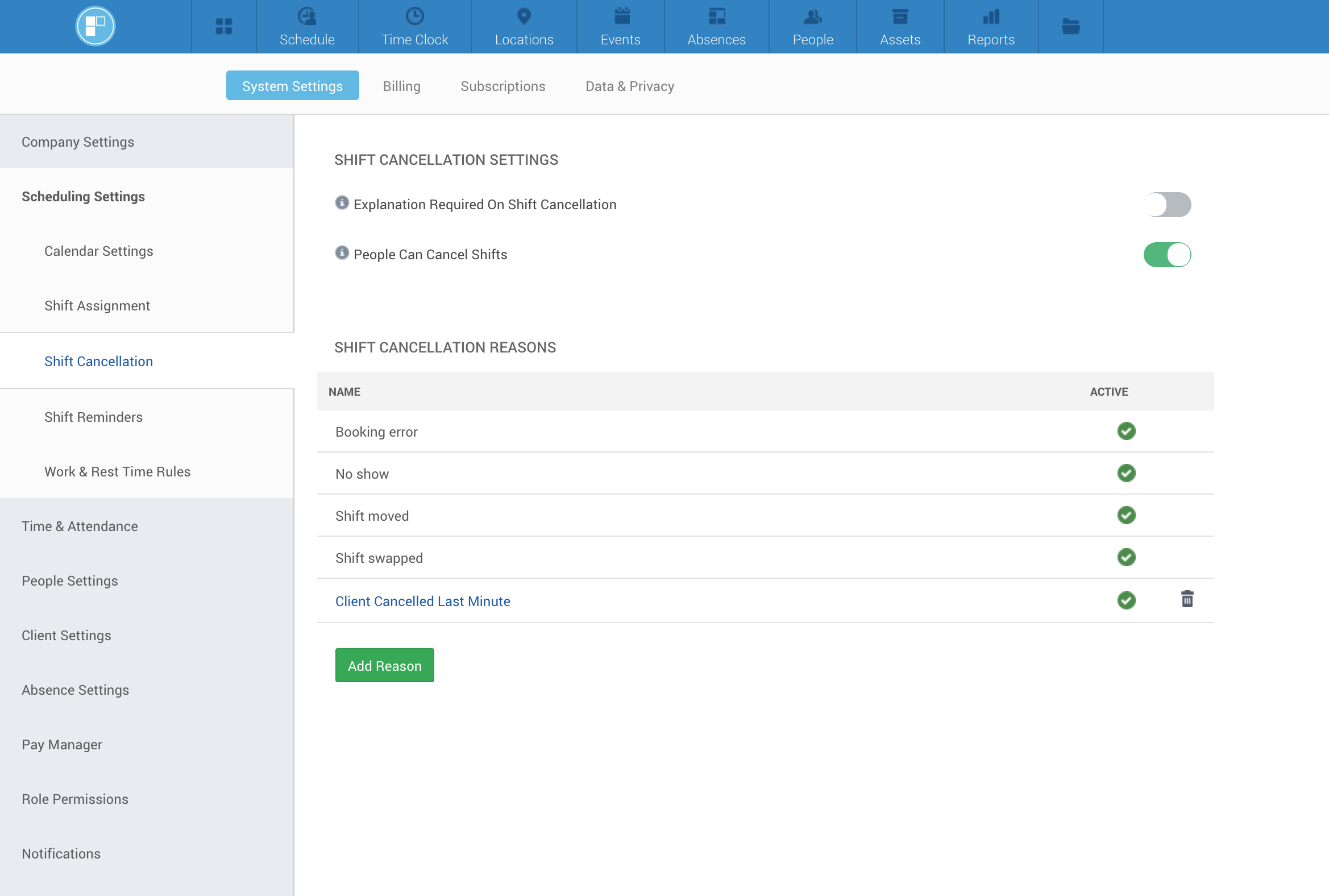The image displays a digital dashboard interface with a blue menu bar spanning horizontally across the top. On the far left of the menu bar, there is a blue square icon with a white symbol resembling a tall coffee cup. Directly beneath this icon is a vertical menu featuring several buttons labeled as follows: "Schedule," "Time Clock," "Locations," "Events," "Absences," "People," "Assets," and "Reports." Additionally, there is an icon resembling a folder without a title.

The screen currently shows the "System Settings" page. Under "System Settings," the first option, "Shift Cancellation Settings," is toggled off, indicating that the detailed explanation required for shift cancellation is not enabled. The next option, "Allow People to Cancel Shifts," is toggled on, signifying that users have the ability to cancel their own shifts.

Below these settings is a list of "Shift Cancellation Reasons," of which the following are checked: "Booking Error," "No Shows," "Shift Moved," "Shift Swapped," and "Client Canceled Last Minute."